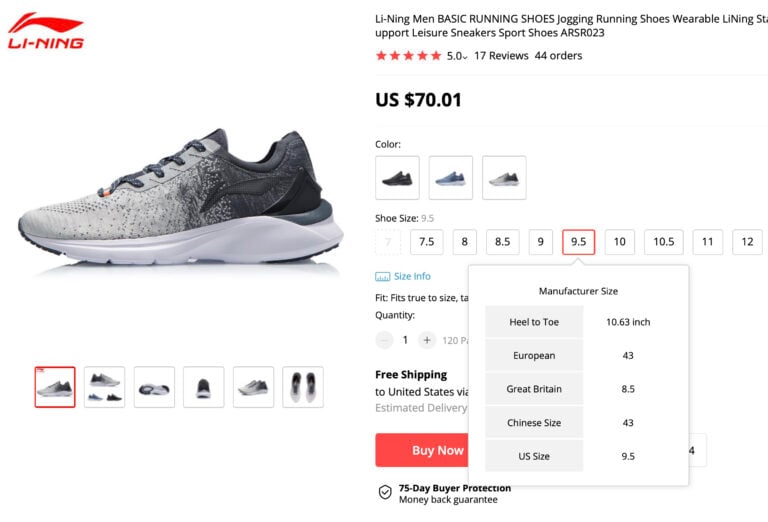Screenshot of Li Ning Website Featuring Men's Running Shoes

The image is a screenshot of a website called Li Ning, captured on a desktop or laptop computer. The upper left corner features the Li Ning logo, showcasing a distinctive red design accompanied by the company name in red, capitalized letters. 

Centered on the page is a product listing titled "Li Ning Men's Basic Running Shoes Jogging Running Shoes Wearable Li Ning Support Leisure Sneakers Sport Shoes SR-023." The product boasts a 5-star rating based on 17 reviews and has been ordered by 44 customers in the past. 

The price is displayed as $70.01 in US currency. Shoppers are presented with three color variations for the sneakers: black, blue, and gray. Available sizes include 7.5, 8, 8.5, 9, 9.5, 10, 10.5, 11, and 12. 

Below the product details, a prominent "Buy Now" button invites users to make a purchase. Additional information about sizes, various product images to browse, and shipping options are provided. The website also highlights a 75-day buyer protection money-back guarantee. 

The screenshot indicates that 120 pairs of these shoes are available for purchase and that the product ships to the United States with free shipping.